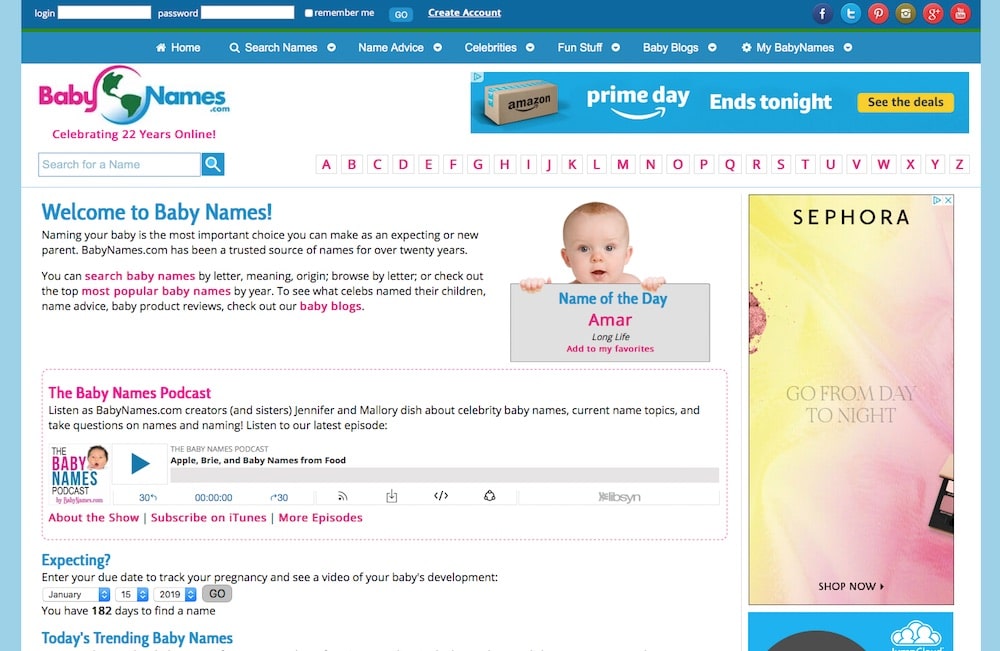The website, babyname.com, features a layout that is wider than it is tall, framed with thin, light blue borders on both the right and left sides. At the top of the page, a dark blue banner encompasses sections for login, password, a 'Remember Me' checkbox, and a 'Go' button. Adjacent to these sections, there is a 'Create Account' link and a series of social media icons.

Beneath the dark blue banner, a thin green line runs across the page, followed by a lighter blue navigation bar. This bar contains tabs labeled 'Home', 'Search Name', 'Name Advice', 'Celebrities', 'Fun Stuff', 'Baby Blogs', and 'My Baby Names', each accompanied by a small icon.

In the upper left area of the website's body, the logo 'babyname.com' is displayed with a distinctive glow effect. To the right of the logo, an Amazon Prime advertisement banner is present. Below these elements, there is a search field for finding names, accompanied by alphabetical buttons for name browsing.

Centered slightly to the left, a 'Welcome to Baby Names' section is highlighted, featuring an image of a baby. Here, various resources are offered, including a baby name podcast, complete with a play button and additional information. 

On the bottom left, a section titled 'Expecting?' allows users to enter their due date, featuring a dropdown to select the date and a 'Go' button. Additionally, there is a segment highlighting trending baby names.

To the right within the body of the website, an advertisement banner for Sheporia is displayed, rounding out the page's content.